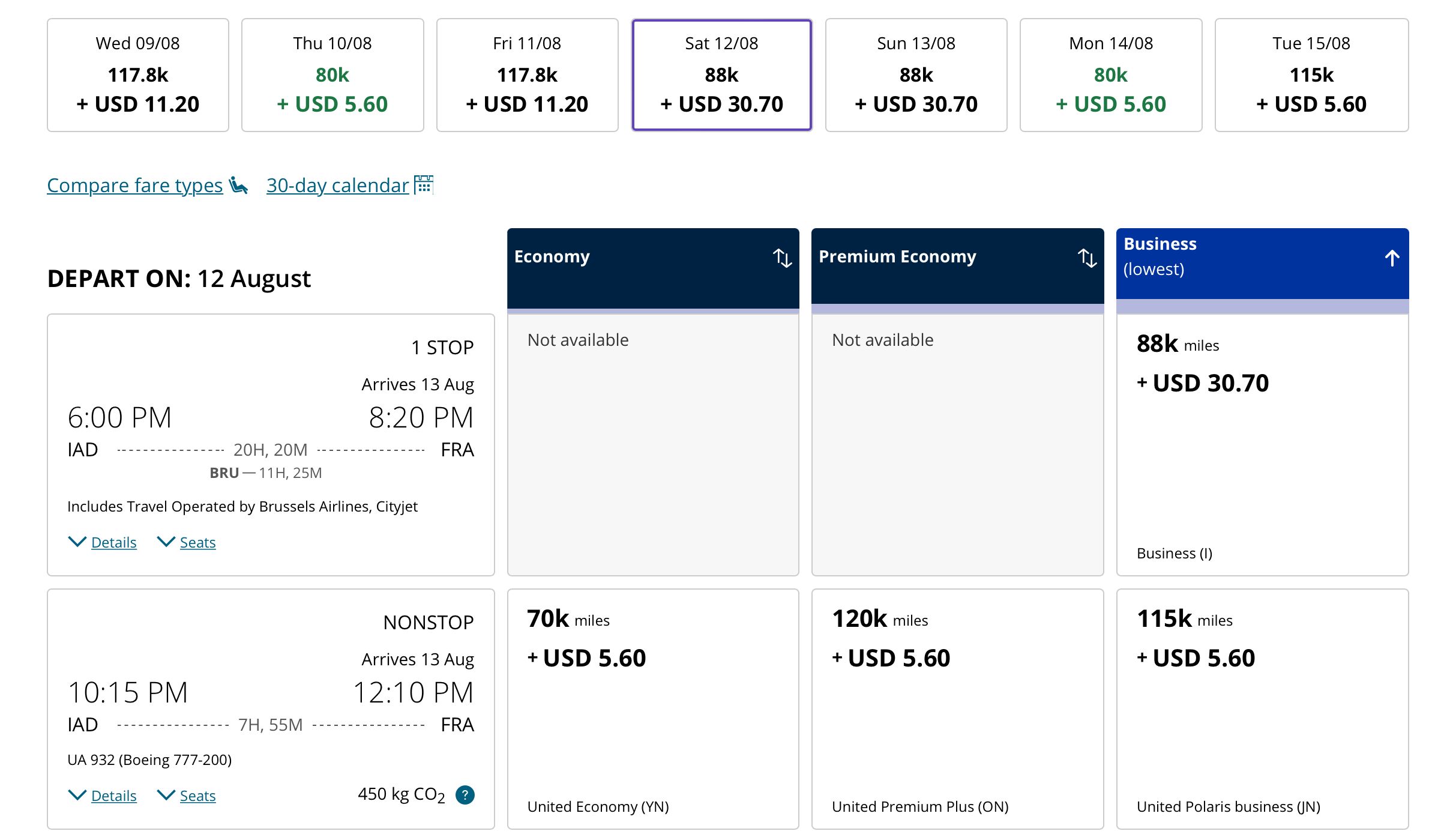The image displays a detailed flight comparison chart, showcasing various flight options sorted by days of the week, with associated costs and details. At the top, there are seven square boxes, each labeled with a day of the week and corresponding data:

1. **Wednesday**: "117,000" miles, "USD 11.20"
2. **Thursday**: "80k" miles, "USD 5.60"
3. **Friday**: "117,000" miles, "USD 11.20"
4. **Saturday**: "88k" miles, "USD 30.70"
5. **Sunday**: "88k" miles, "USD 30.70"
6. **Monday**: "80k" miles, "USD 5.60"
7. **Tuesday**: "115,000" miles, "USD 5.60"

Underneath these boxes, there's a section for comparing different fare types over a 30-day calendar. The details include a departure window from 6:00 PM to 8:20 PM with one stop, likely indicating flight duration and layovers.

The flight comparison is intended to help users select optimal flight dates based on miles and cost. For example, flights on certain days might cost an additional "USD 11.20" or "USD 30.70" if opted for.

The flight is scheduled for August 12th, traveling from IAD (Washington Dulles International Airport) to FRA (Frankfurt Airport). The top section of the chart categorizes flights into "Economy", "Premium Economy", and "Business", indicating that the user might be considering booking a "Business" class ticket given the context and details reviewed.

Overall, it appears to be a comprehensive flight booking page allowing users to compare prices and dates effectively, facilitating an informed decision on travel plans.